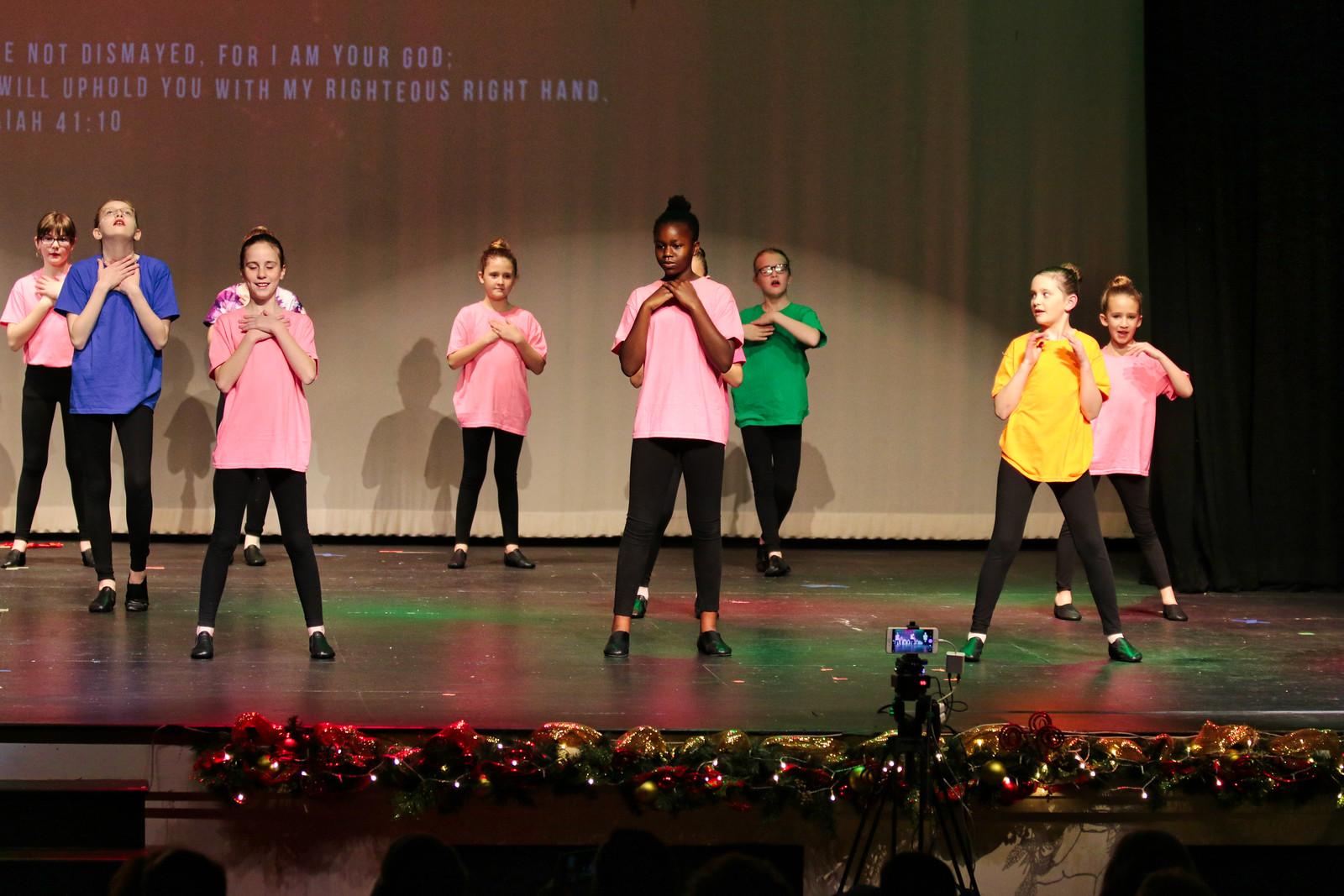This detailed photograph captures a children's dance performance taking place on a stage adorned with a white curtain backdrop partially displaying the words, "Do not be dismayed, for I am your God; I will uphold you with my righteous right hand. 4110." The stage features several young dancers, including one Black girl and several white girls, all wearing identical black leggings and shoes. Most of them are dressed in pink t-shirts, while others stand out in blue, green, and yellow t-shirts. The dancers hold their hands crossed around their necks, poised to begin their performance. Below the stage, a camera on a tripod is set up, possibly recording or photographing the event. Additionally, a festive garland with lights and ribbons decorates the front of the stage.